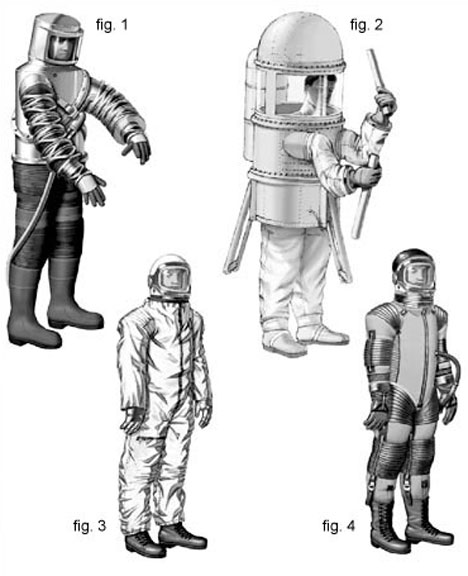This is a detailed black and white 1960s-style illustration depicting four vintage spacesuit designs, each worn by a figure and annotated with a figure number. Figure one features a man clad in rubber boots, a metal jacket, and a clear helmet, with wires wrapped around his arms, allowing visibility. Figure two shows a man in a more cumbersome, dome-shaped suit resembling an enclosed metal tube; he holds a pipe in each hand. Figure three represents the simplest design, a one-piece spacesuit with a helmet, offering minimal bulk. Figure four displays a full-body suit in gray and white, striking a balance between flexibility and enclosure. The figures mostly stand still, except for one, adding dynamism to the illustration.